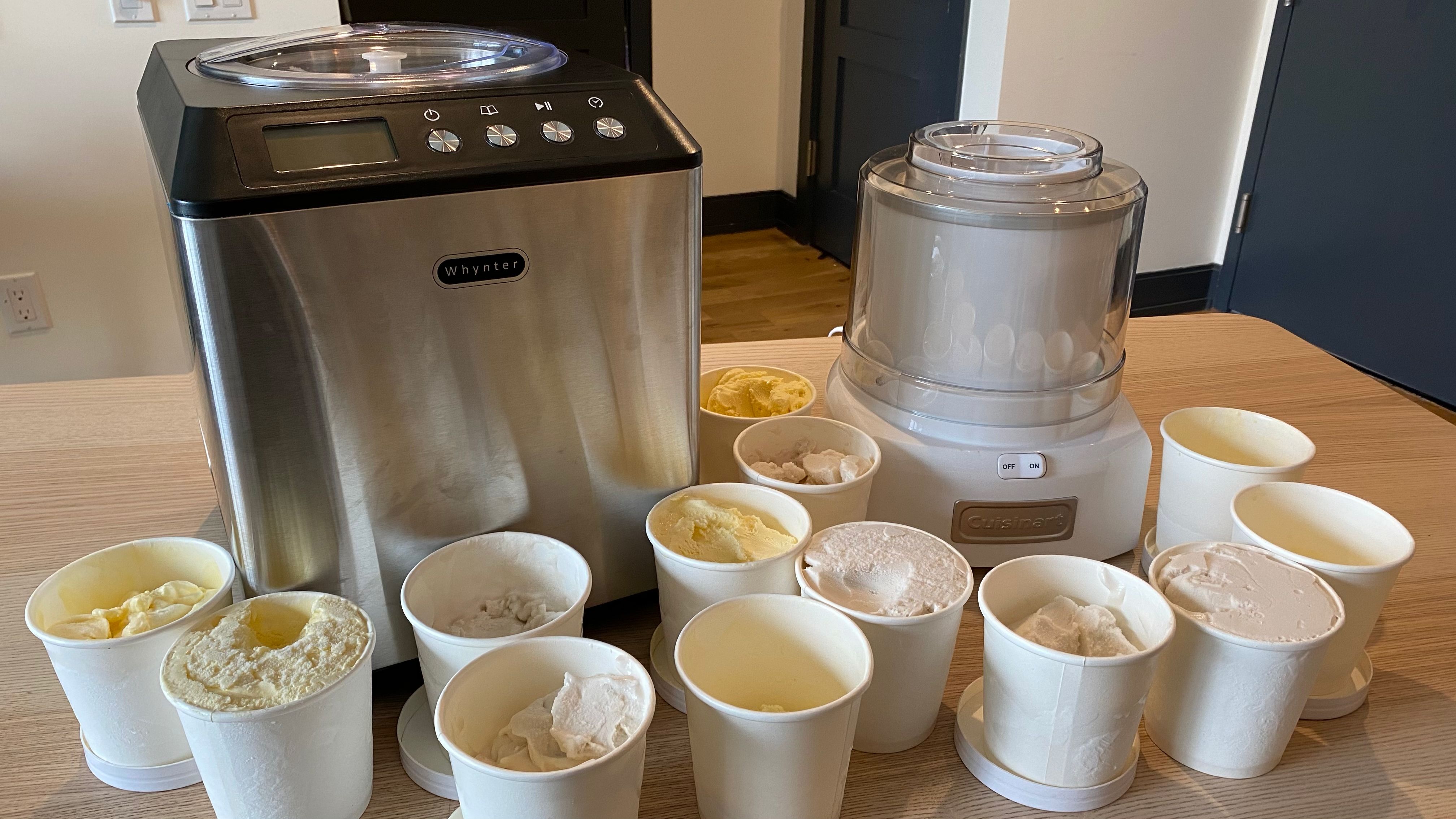In a cozy indoor setting, this image captures a bustling kitchen scene featuring a light-colored wooden table. The table, which appears to be in either an office or a home, is situated in front of white walls with black trimming and dark blue or black doors in the background. The countertop is adorned with two conspicuous machines. On the left, there’s a large, rectangular silver machine branded with the name "Whynter," complete with a black top, silver buttons, view screen, and a circular white lid. To its right is a smaller white Cuisinart machine, featuring a circular top with a small opening.

Surrounding these machines are approximately thirteen paper cups, possibly more, each placed with their lids nearby. These cups seem to contain homemade ice cream in various light colors, some whitish while others have a yellowish tint. There are electrical sockets visible on the left side of the image, indicating that this could be an experiment or preparation of different flavored ice creams to be frozen for later consumption, set against the backdrop of brown wood flooring.